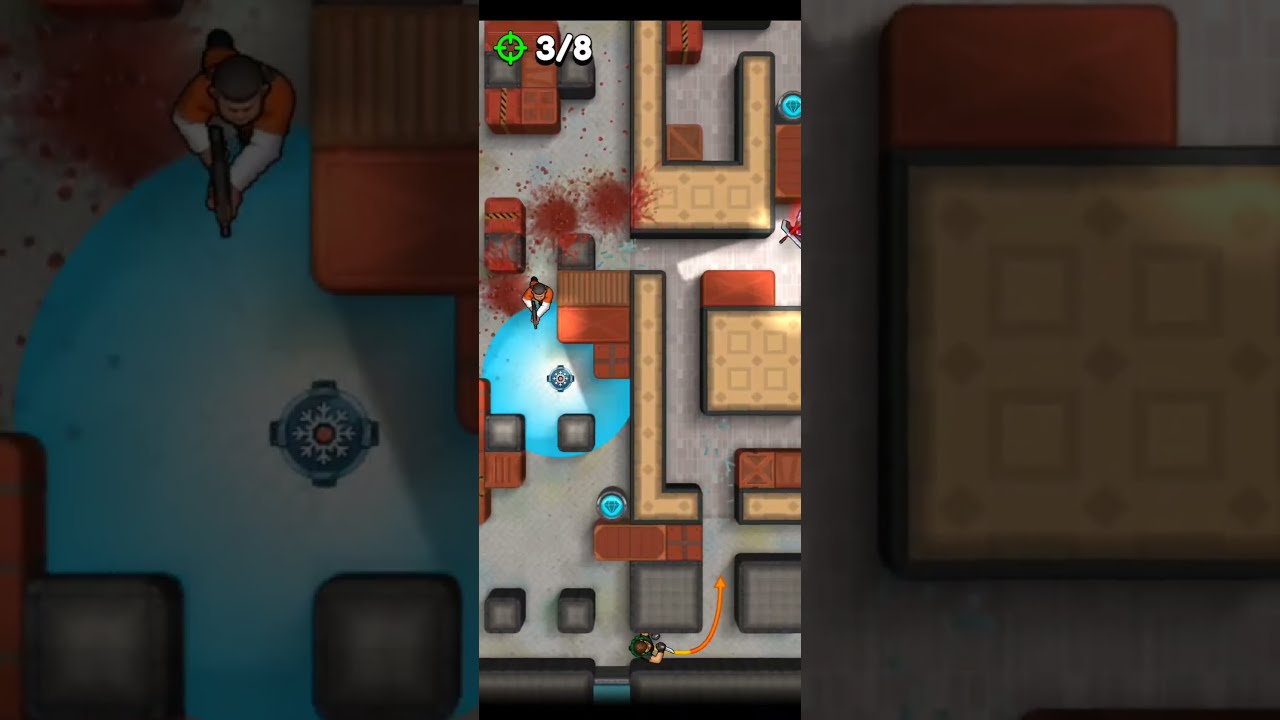This image is a detailed screenshot from a top-down shooter video game, presented in a three-panel horizontal format, where the left and right panels are close-up views of the center image from different angles. The central panel showcases an aerial view of a small town-like maze filled with tan L-shaped walls, gray squares, and scattered brown crates. In the bottom middle of this panel, a character wearing a green shirt is visible, positioned between a wall and another structure, with a looping orange arrow indicating his path. Above him, there is a figure in an orange shirt wielding a black gun, with noticeable blood splatters on the concrete beneath. The left and right panels magnify the center section, emphasizing the presence and detailed textures of the maze, characters, and evident bloodstains. The scene captures the tense moments of the game, highlighting the player's challenge as they navigate through the maze, potentially trying to evade the armed individual. The score displayed in the game is 3 to 8, adding context to the competitive nature of the scenario.